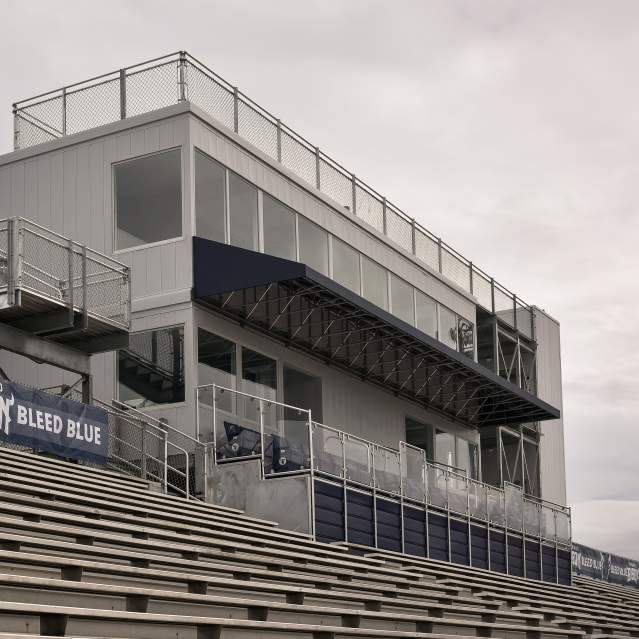The image captures a cloudy-skied outdoor stadium, focused on a section of bleachers and an adjacent two-story building. The bleachers, composed of stone or grey material, are arranged in a descending order from the top of the image. On the left side, a prominent blue banner with white lettering reads "Bleed Blue," advocating team spirit. Below this banner, there are several benches that descend downward into the general admission area. To the right at the bottom, barely visible, there are some advertising signs and pull-down slat doors which likely serve as vendor or storage spaces.

Above the bleachers, a two-story structure is revealed, featuring multiple panes of glass arranged horizontally, suggestive of a corporate box or loges for spectators. This area is partially covered by a blue metal roof, shielding two rows of outdoor seating, which are separated by glass and metal railings. The building is accompanied by stairs leading up to different seating levels and is surrounded by greyish panels and chain-link fences. This intricate setup ensures both private and general viewing spaces, creating a comprehensive view of this stadium section.